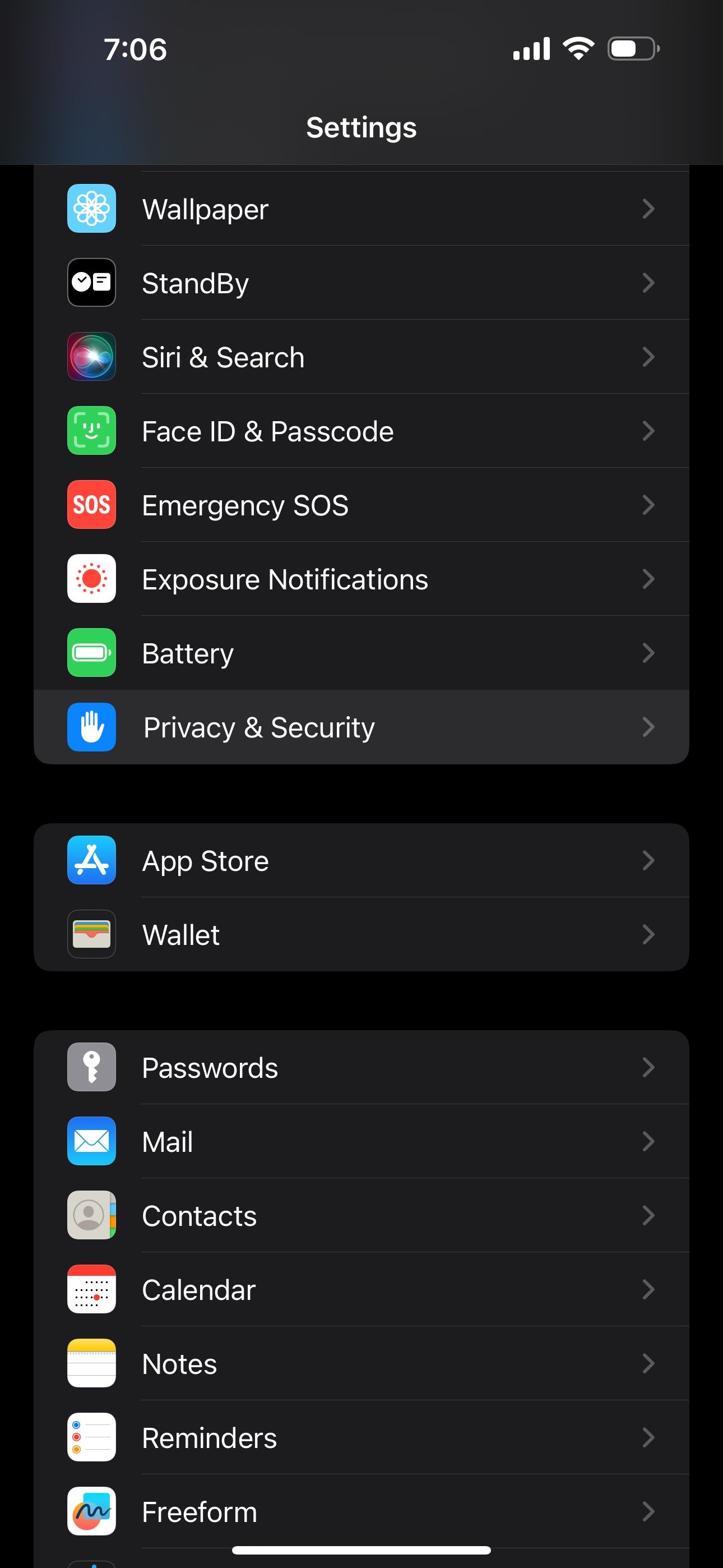This image captures a screenshot of an iPhone displaying its Settings page, set against a sleek black background indicative of the device’s dark theme setting. At the top left corner, the time is clearly shown as 7:06. The top right corner boasts a full network signal with 4 out of 4 bars, a WiFi signal strength of 3 out of 3 bars, and a battery level indicator displaying ample charge. On the main screen, a variety of settings options are visible in a scrollable menu. These include familiar categories such as "Wallpaper," "Standby," "Siri & Search," "Face ID & Passcode," "Emergency SOS," "Exposure Notifications," "Battery," "Privacy & Security," "App Store," "Wallet," "Passwords," "Mail," "Contacts," "Calendar," "Notes," "Reminders," and "Freeform." Below these settings options, the iPhone’s navigation bar is also visible, seamlessly blending with the dark theme aesthetic.